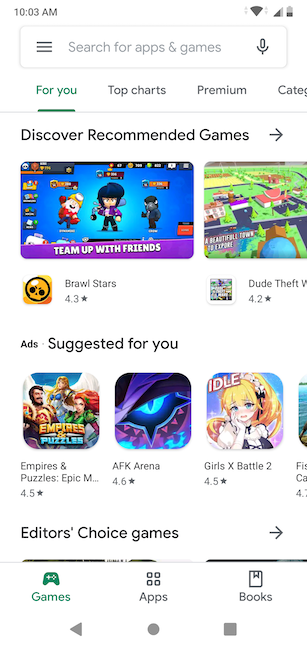This image is a screenshot captured from the Google Play Store interface at 10:03 AM, as indicated by the black timestamp at the top. The status bar displays a Wi-Fi symbol and a battery icon. Below, a white search box features three black lines, a black microphone, and the prompt "Search for apps & games."

Scrolling down, several submenus are displayed: "For You" is highlighted in green, while "Top Charts," "Premium," and "Categories" are shown in gray. 

Further down, the section "Discover Recommended Games" is in black text, accompanied by a rightward arrow. The first game, "Brawl Stars," rated at 4.3 stars, showcases a screenshot with the phrase "Team Up with Friends" in white and purple text. The image includes cartoon icons: a small white character in a yellow hat and red shirt waving, another character with blue hair dressed in purple and black holding an 8-ball, and a gray character in a blue jacket and black pants.

Following that, another game named "Dude Theft," rated 4.2 stars, features a colorful city map with shades of pink, green, and tan, along with visible roads. 

The section "Ads Suggested for You" highlights several games with their accompanying graphics:

1. "Empires & Puzzles," rated 4.5 stars, features a red-headed woman in green, a blonde woman in a blue top, and a man with brown hair and facial hair dressed in gold-red armor. The game title is split with "Empires" in orange and "Puzzles" in blue.

2. "AFK Arena," rated 4.6 stars, shows a partial eye and face view of a dragon in purple, blue, pink, and black tones.

3. "Girls X Battle 2," rated 4.5 stars, displays an anime-like character with pale white skin, blond hair embellished with a black-and-white accessory, wearing a black and white dress, with one hand under her chin. 

A partial water scene from another game is visible below this section. 

At the bottom of the image, "Editor's Choice Games" is highlighted next to a green game controller icon. The navigation bar shows icons for "Games" (four black squares), "Apps" (a book icon), "Books," and the standard Android navigation icons: a triangle, circle, and square.